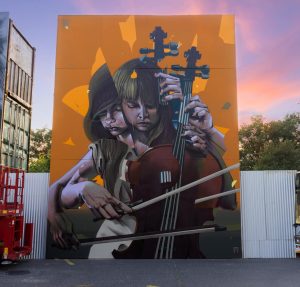This image showcases a striking, large mural on a corrugated metal panel, potentially part of a shipping crate, awaiting placement. The mural features an intricate and non-photorealistic depiction of a young girl and an older woman, both playing a violin. The design is fragmented, with multiple heads and several arms emerging, holding bows that intricately cross the violin’s strings, creating a surreal, dynamic effect. The main figures have dark brown hair, with the younger girl’s hair styled with bangs, and their expressions are focused downward. The background of the mural is primarily deep orange with occasional bright orange fragments, enhancing the vibrancy of the scene. The setting also includes a forklift to the left, a corrugated metal fence, green leafy trees, and a sky tinged with sunset hues of pink, purple, and blue, making for a visually captivating and complex artwork.